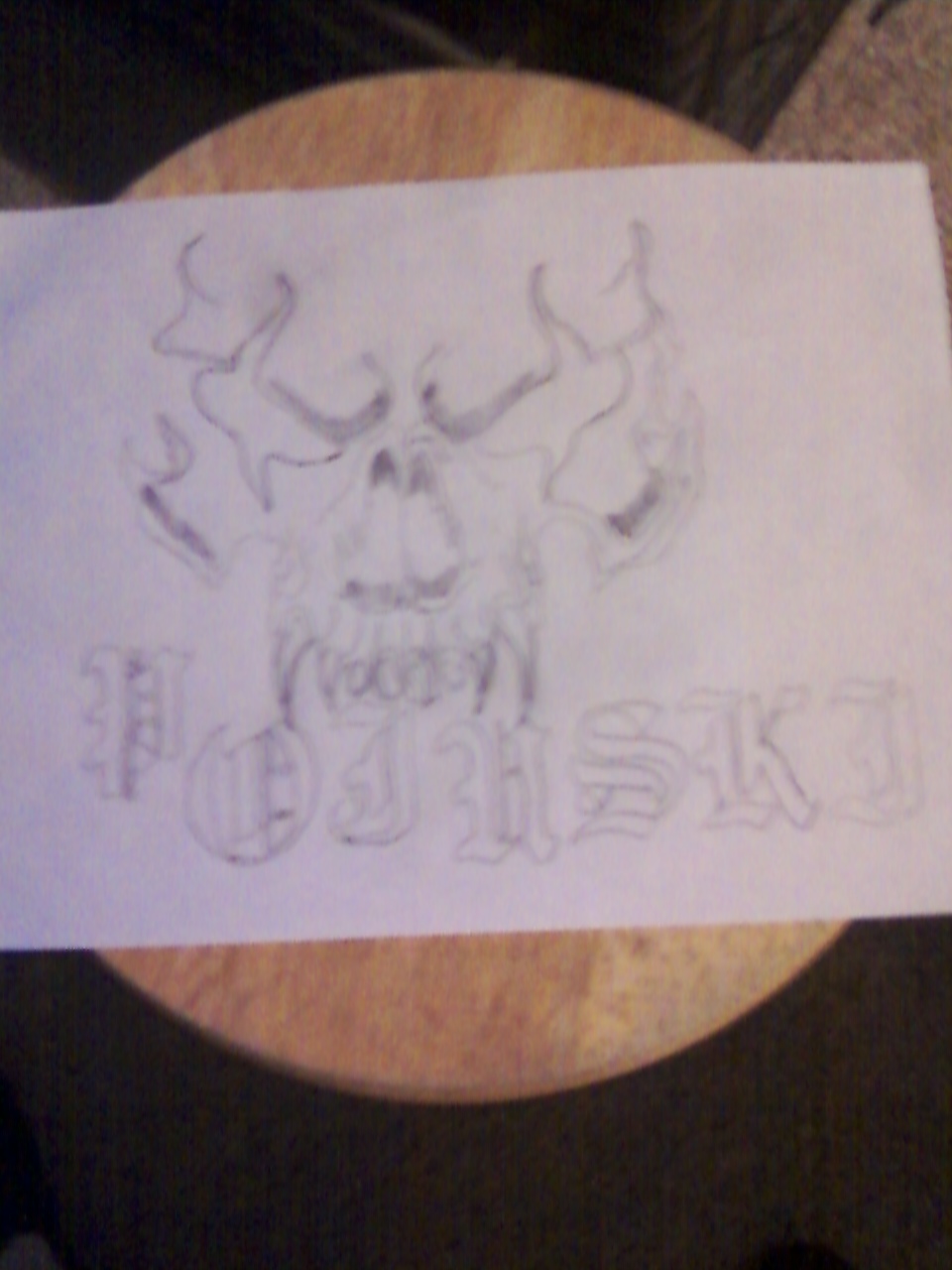The photo, albeit out of focus, depicts a hand-drawn illustration on a plain rectangular piece of paper, oriented horizontally. This paper is placed atop a round wooden stool, with a section of carpet visible in the top-right corner of the image. The drawing itself appears to have been created using either pencil or marker, and features a detailed skull, complete with prominent teeth, a nose cavity, and a jaw structure. Beneath the skull, there is a string of letters that include "P," "O," "H," "S," "K," and either an "I" or a "J," though the exact sequence is somewhat obscured.